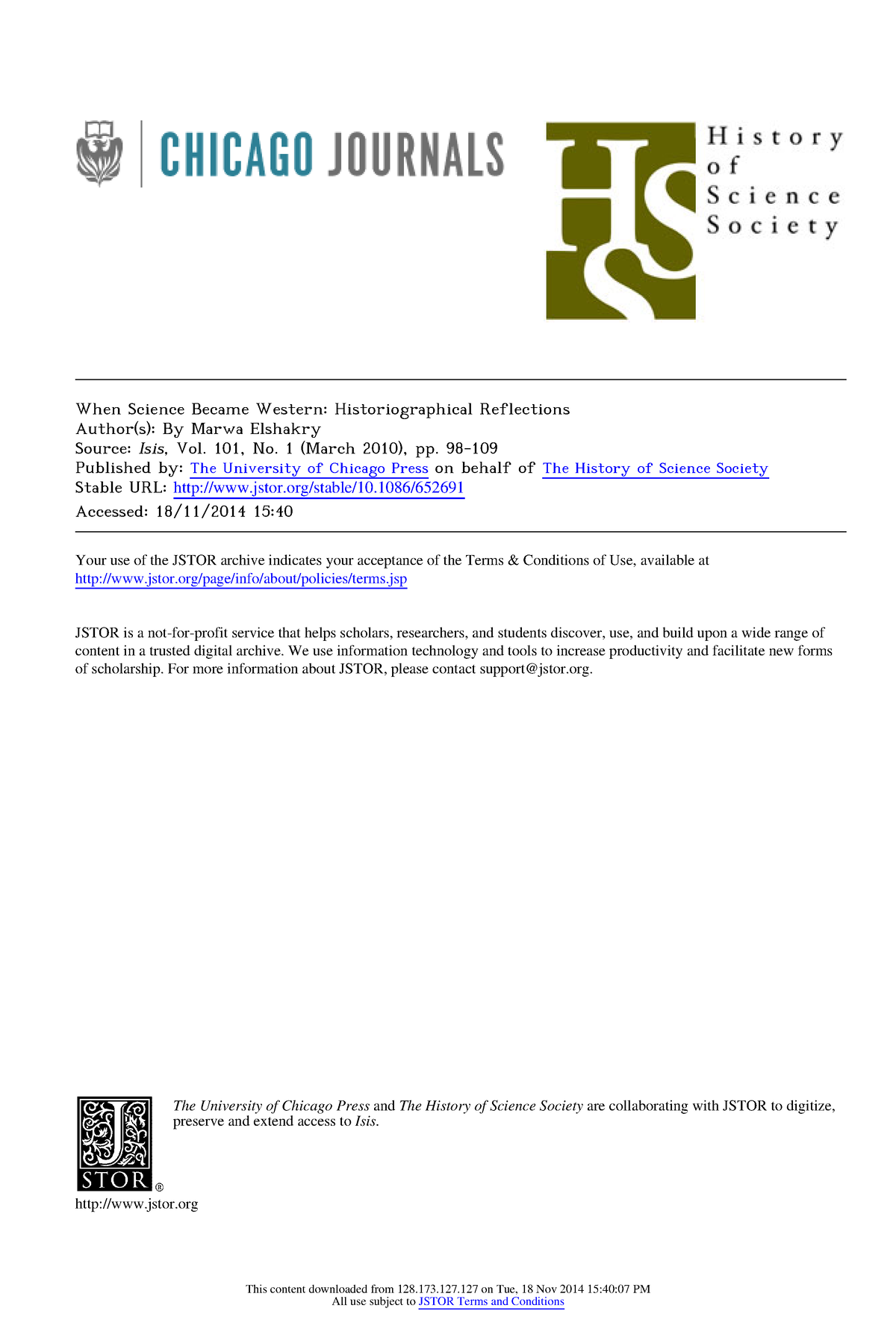The image is a screenshot from a website, displaying various elements related to the Chicago Journals. In the top left corner, there's a logo featuring a coat of arms, followed by a small vertical gray line. Adjacent to this line, the text "Chicago Journals" is displayed, with "Chicago" in teal and "Journals" in dark gray. 

On the top right corner, there's a large, portrait-oriented rectangle containing the letters "HSS" in a khaki green color. Alongside this block, the text "History of Science Society" is positioned. All of these elements are underscored by a thin black line.

Below this line, in an exceptionally small font, the text begins with "When Science Became," but the remainder is nearly illegible. It continues with "Something Historiographical Reflections, authored by [Author’s Name], source, and then published by," followed by a link to the University of Chicago Press on behalf of the History of Science Society. It also includes a stable URL for the book, noting it was accessed on 18-11-2014 at 15:40. 

Another thin black line runs underneath this section. Below this second line, additional information is provided, including a segment in italics that appears to be a disclaimer or a note.

Towards the bottom of the image, near the left side, there's a beautifully stylized "J" accompanied by some related information. At the bottom center of the image, there's small print likely containing details pertinent to the web page itself.